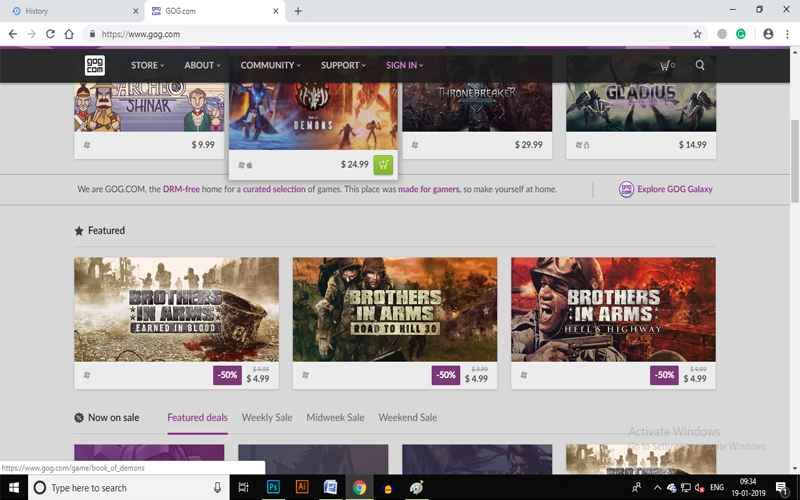This screenshot captures the homepage of GOG.com, a website known for offering DRM-free video games. The address bar prominently displays "https://www.gog.com," indicating secure access to the site. Just below, the site's navigation menu features a GOG.com logo, followed by options for browsing a drop-down menu labeled "Store," "About," "Community," and "Support," along with a sign-in button on the far right.

Beneath the navigation menu, four game thumbnails are prominently displayed, likely highlighting featured or popular games. Each thumbnail includes pricing information: the first game is priced at $9.99, the second at $24.99, the third at $29.99, and the fourth at $14.99. The visual layout suggests a user-friendly interface, designed to quickly catch the visitor's eye and guide them through their gaming selections.